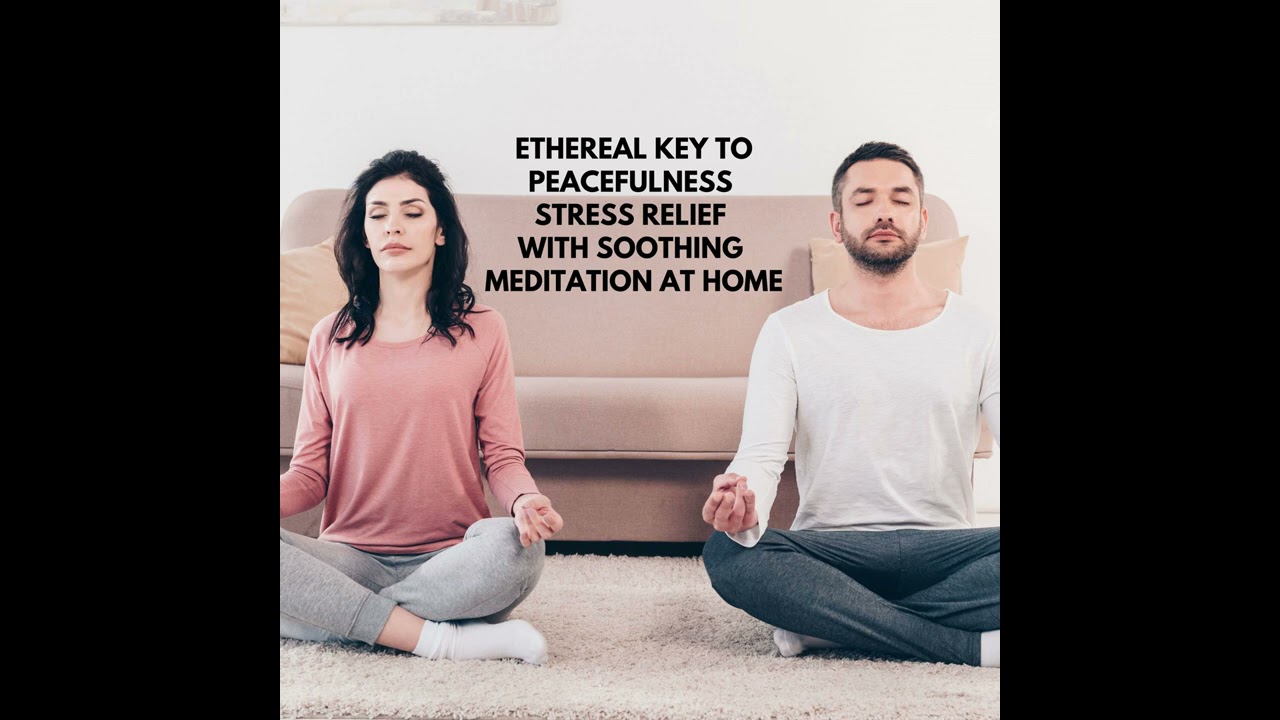The image portrays a serene scene of a couple meditating in their home, set against a stark contrast with black panels on either side of the rectangular frame. The couple sits on a plush white shag carpet in front of a tan couch and a white wall, exuding a tranquil atmosphere. The woman on the left, with long dark hair, wears a muted salmon pink blouse, gray sweatpants, and white socks, and sits with her legs folded under her in a traditional meditative pose. Her partner on the right, a man with short brown hair and a light beard, mirrors her posture. He dons a loose-fitting white top and dark gray pants. Both have their eyes closed, deeply immersed in meditation. The ambiance is accentuated by the text overlay in black, reading: "Ethereal key to peacefulness, stress relief, with soothing meditation at home." The overall tone is one of calm and introspection, emphasizing the peaceful benefits of meditation.